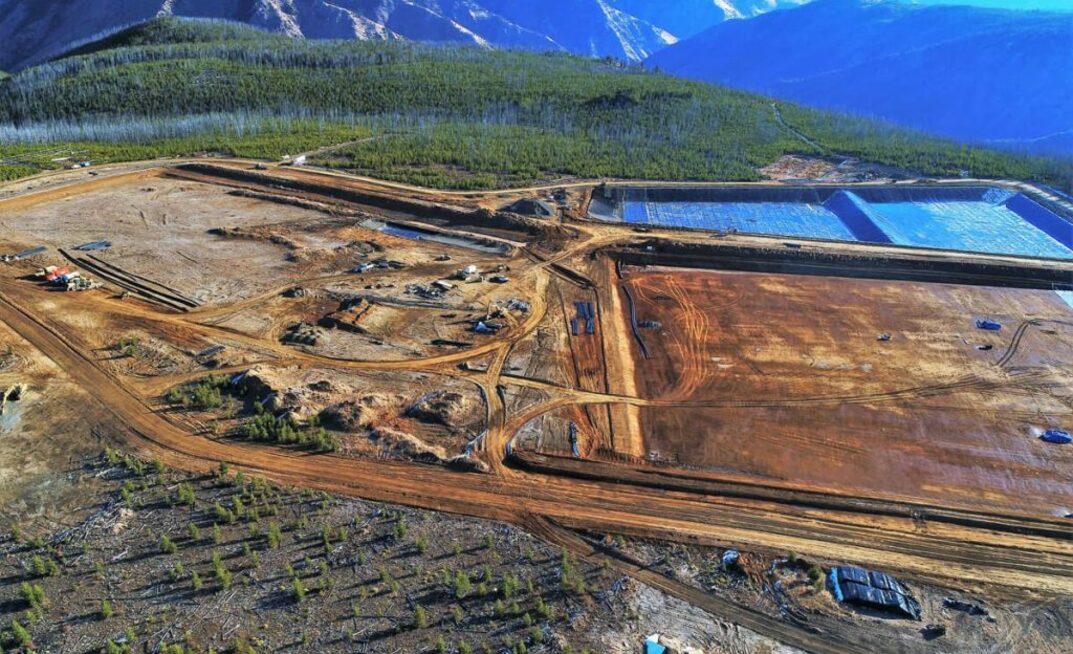This aerial photograph, possibly taken from a helicopter or airplane, offers a comprehensive overview of a sprawling, excavated mining area nestled within a forest landscape. At the top of the image, distant mountain ranges exhibit gray tones on the left and blue hues to the right. Below these ranges, grassy and hilly terrain spans the image, interspersed with patches of white vegetation.

Dominating the center of the photo is an extensive expanse of brown, excavated ground. This area features a network of dirt roads crisscrossing the scene, with one prominent road running from the middle left to the lower right. To the right of this main thoroughfare lies a large brown field, largely barren but punctuated by a few scattered vehicles, hinting at ongoing or preparatory mining activities. Adjacent to this are two blue, pool-like structures separated by a vertical blue divider and bordered by white walls, their purpose unclear but reminiscent of large swimming pools.

On the higher left side of the image, notable gray dirt contrasts with structures amidst rocks and trees, alongside visible vehicles and equipment, likely used for excavation. Scattered throughout the scene are various vehicles, including trucks in red, blue, white, and tan, signifying active industrial operations.

At the bottom of the photograph, the landscape transitions into areas of open dirt, mingling with occasional trees particularly visible on the left. The leftmost section also displays a mixture of green and yellow grass and some scattered black and blue elements. Overall, the image vividly captures the interplay between industrial activity and natural elements in this dynamically altered wilderness area.